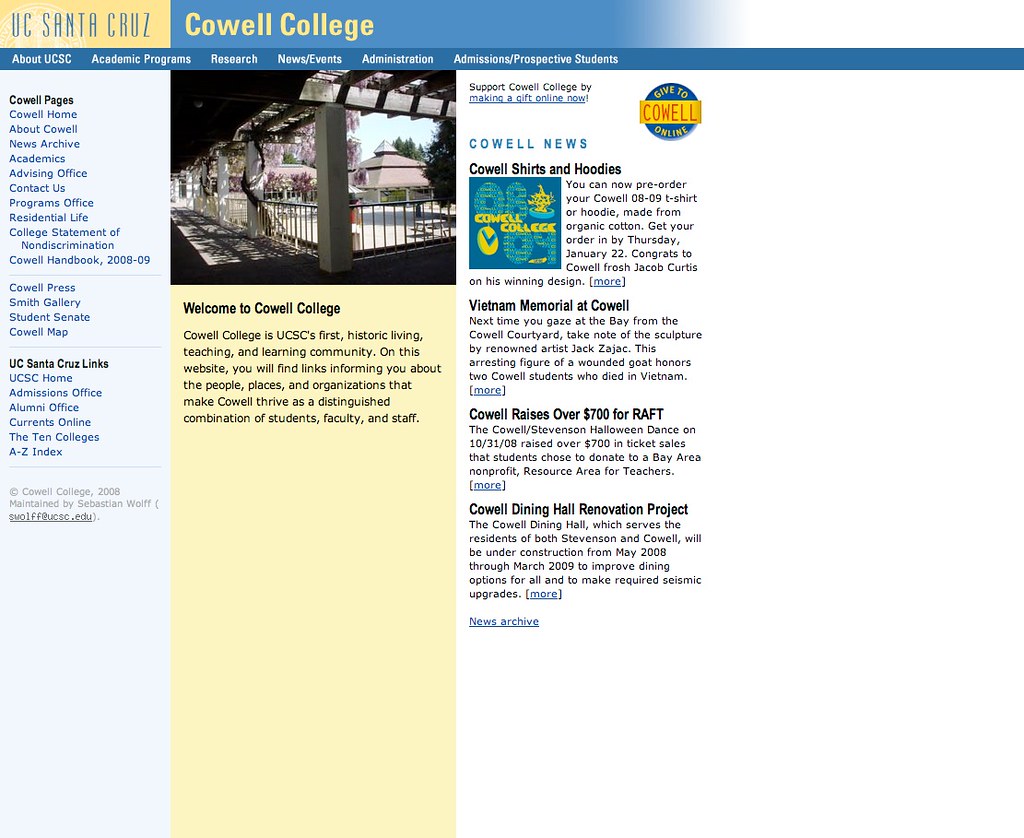The image depicts a webpage from the University of California, Santa Cruz (UC Santa Cruz) website, dedicated to Cowell College. In the top left corner, there is a small yellow banner that reads "UC Santa Cruz." Adjacent to this, extending towards the center, is a blue banner that fades into white, featuring the text "Cowell College" in yellow print.

Below these banners, a long blue horizontal section spans across the webpage with navigational links including: "About UCSC," "Academic Programs," "Research," "News/Events," "Administration," and "Prospective Students." 

On the left side of the page, there is a vertical menu listing Cowell-specific pages: "Cowell Home," "About Cowell," "News Archive," "Academics," "Advising Office," "Contact Us," "Programs Office," "Residential Life," "College Statement of Non-Discrimination," "Cowell Handbook," "Cowell Press," "Smith Gallery," "Student Senate," and "Cowell Map." 

Additionally, a section labeled "UC Santa Cruz Links" provides quick access to: "UCSC Home," "Admissions Office," "Alumni Office," "Currents Online," and an "A to Z Index" of the 10 UCSC colleges.

Centrally located on the webpage is an image of an outdoor scene featuring campus buildings and blooming flowers. Beneath this image, text welcomes visitors to Cowell College and provides information about the college and its staff.

On the right side of the page, there is a call-to-action, encouraging visitors to support Cowell College by making a gift online, followed by updates under a "Cowell News" section.